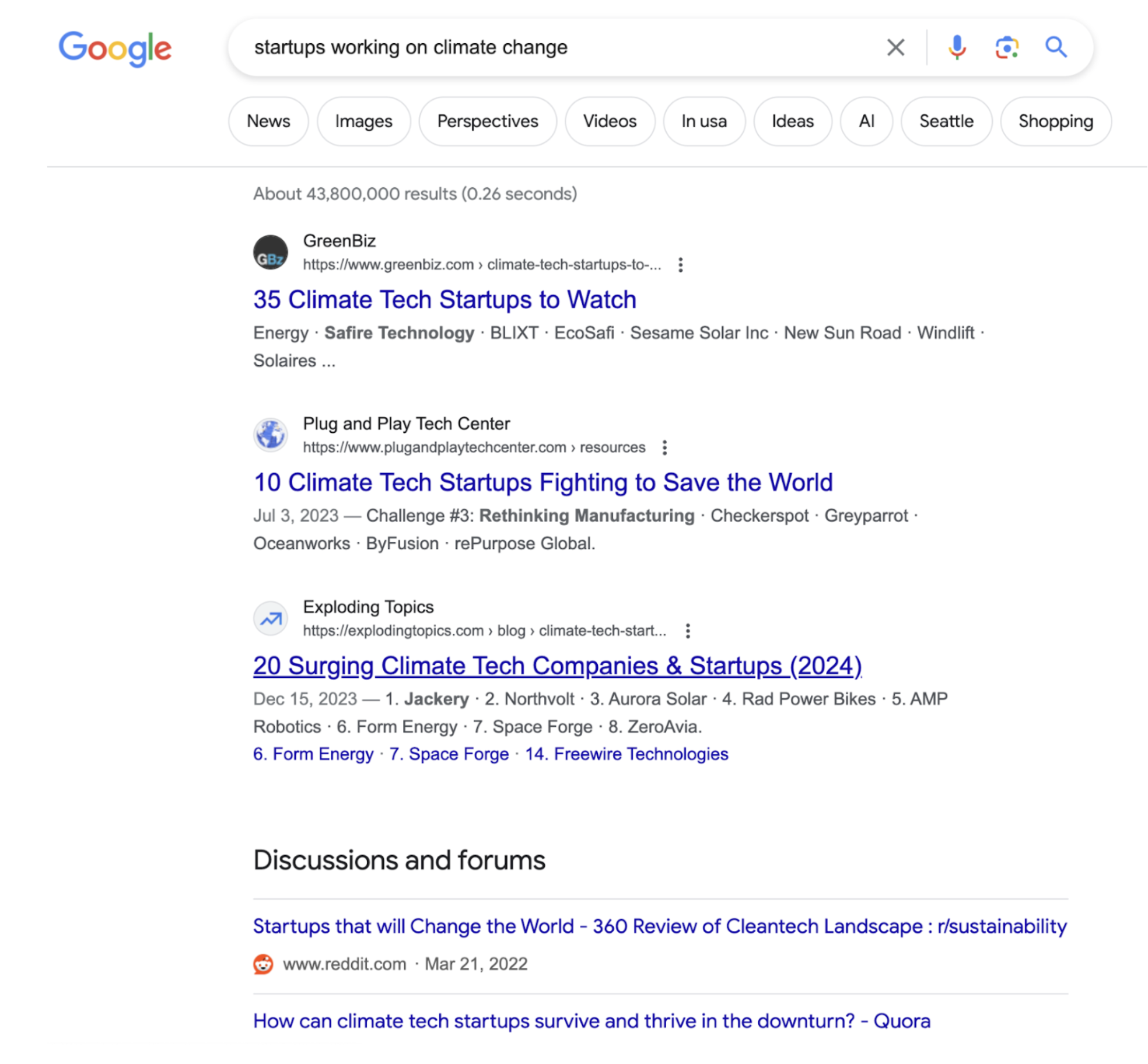A detailed caption for the given image could be:

"The image displays a Google search results page with the word 'Google' prominently featured in its signature four colors— blue 'G', red 'O', yellow 'O', blue 'G', green 'L', and red 'E'— in the upper left corner. Below the logo lies the search bar with the query 'startups working on climate change' typed in. Adjacent to the search bar on the right, there is a microphone icon for voice searches, followed by an enigmatic icon of a dot within a square whose function is unclear, and finally a magnifying glass icon to initiate the search.

Underneath the search bar, various sub-search categories are available in the form of white buttons with black text and grey outlines against a white background. These categories include News, Images, Perspectives, Videos, USA, Ideas, AI, Seattle, and Shopping. 

The main content of the page indicates that there are approximately 43,800,000 results found in 0.26 seconds, with initial search results focusing on climate tech startups prominently displayed.